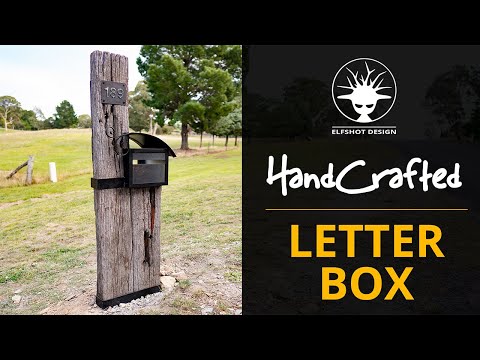This image is an advertisement for Elfshot Design, featuring a handcrafted letterbox. The background is predominantly black, with the advertisement text on the right-hand side and an inset photograph to the left. At the top of the advertisement, the text "Elfshot Design" is accompanied by a circular logo of an elf-like creature's head with antlers and pointed ears. Below the logo, the word "handcrafted" is written in white, underscored by a yellow line. Beneath this line, the word “letterbox” appears in mustard yellow text.

The inset photograph, located on the left side of the image, depicts an outdoor country scene with a grassy field and a few trees in the background. Central to the photo is a wooden post, bearing a plaque with the street number "189." Attached to this post is a black letterbox, presumably the product being advertised. The wood of the post appears oak-aged, contributing to the rustic and handcrafted aesthetic that the company emphasizes. The advertisement clearly highlights the product’s use as a mailbox for residential driveways, appealing to those looking for unique, handcrafted mail solutions.